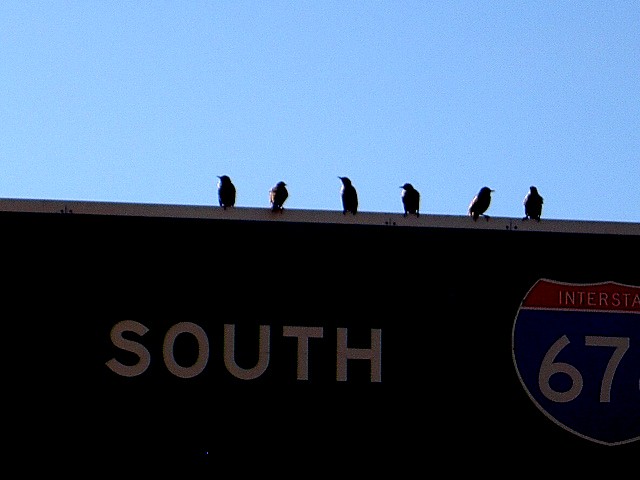In this detailed photo taken in daylight, against a clear blue sky backdrop, an interstate sign prominently fills the frame. The sign, colored green with white lettering, reads "South Interstate 67." The distinctive interstate shield, featuring a red top section with the word "INTERSTATE" in white, and a blue bottom section showcasing the number "67" also in white, is clearly visible. Perched atop the sign are six small birds, likely finches or magpies, their silhouettes stark against the bright sky. The birds, casting small shadows, have short black beaks and appear in various orientations—some looking left, others right, and a few directly ahead. This image captures the serene randomness of nature intersecting with human infrastructure.